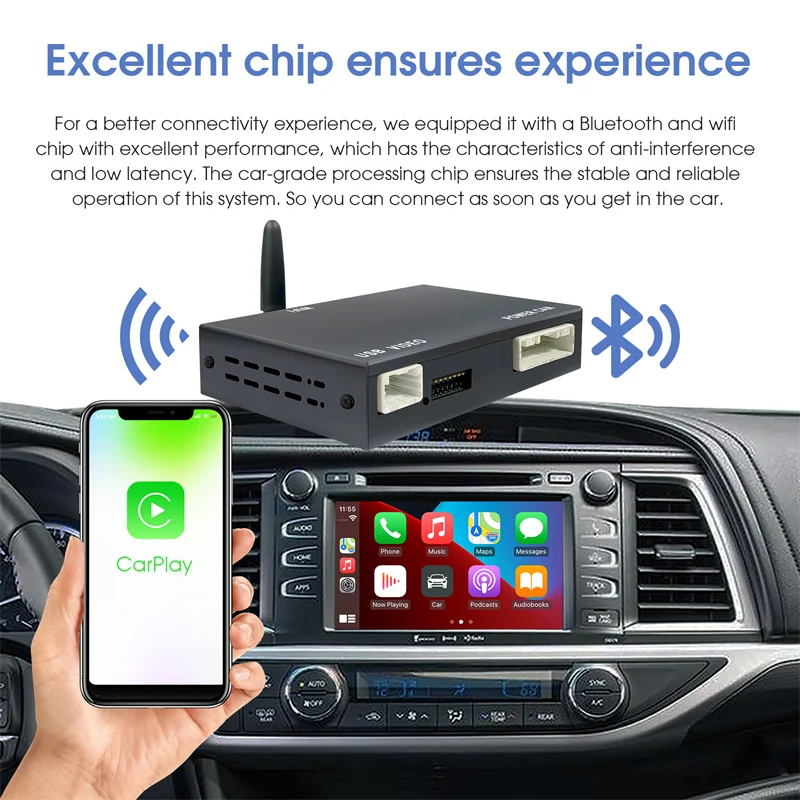This image is an advertisement for a CarPlay product, prominently featuring a robust car grade processing chip for superior connectivity. The top of the image showcases a bold blue text that reads "Excellent Chip Ensures Experience," followed by a descriptive paragraph in black text. The paragraph highlights that the product is equipped with a Bluetooth and Wi-Fi chip known for its excellent performance, anti-interference capabilities, and low latency, ensuring stable and reliable operation as soon as you enter the car.

The visual elements include a hand holding a smartphone displaying the CarPlay logo and business name in green. Central to the photo is the car's infotainment system situated within a black dashboard, featuring a rectangular screen displaying the Apple CarPlay interface. Positioned above the dashboard is the featured product, a black rectangular box with an attached antenna, illustrating its role as a modem for connectivity. The Bluetooth and Wi-Fi icons appear in blue on either side of this device, reinforcing the connectivity features. The entire setup is designed to emphasize the seamless connectivity experience provided by the CarPlay product.